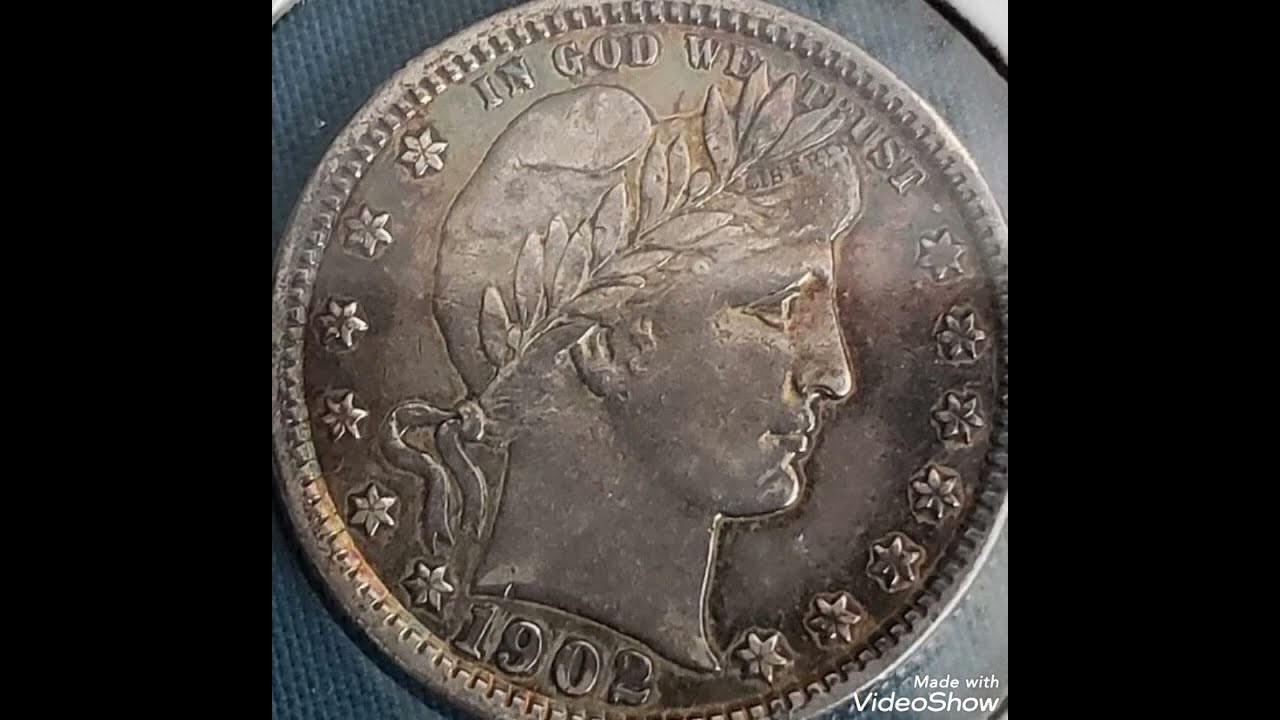In this high-resolution photograph, the central focus is a weathered, silverish-gold coin prominently displayed against a blue textured background. The coin, marked with the year "1902," showcases intricate details including a circlet of stars around its edge, akin to a floral pattern with six-point petals. It features the side profile of a head, likely representing Lady Liberty, adorned with a wreath of leaves that resembles a fig leaf and has the word "LIBERTY" inscribed on a banner across it. The phrase "IN GOD WE TRUST" is engraved at the top. The border of the image includes black vertical rectangles on each side, enhancing the framing of the coin. In the bottom right corner, white text reads "Made with Video Show," highlighting the origin of the photo. The entire composition appears to be part of a personal coin collection, given its meticulous presentation and detail.